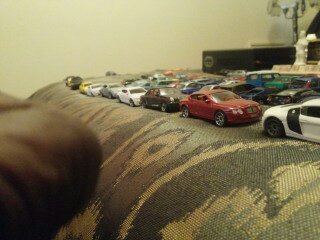The image depicts a collection of small toy cars meticulously lined up on a textured bedspread that features black, cream, and light green hues. The toy vehicles include a diverse assortment of models, such as sports cars, sedans, luxury saloons, and even what appears to be a small truck or jeep. The photo, which has a notable yellow tint and low contrast, shows the cars organized in various ways, with some forming neat rows and others arranged in a more haphazard manner, reminiscent of an organized junkyard. The bedspread spans the entire surface of the bed, with cars stretching from one edge to the other. In the background, a beige-colored wall and a lamp on a small stand are visible, while in the foreground, an elbow and possibly a knee appear, hinting at the presence of a person who might have painstakingly arranged the toys for display.